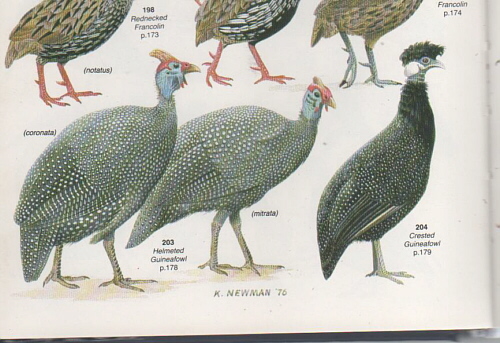This image appears to be the bottom half of a page from a 1975 bird field guide with pen and ink drawings by K. Newman, showcasing three different guinea fowl species. The page includes a crested guinea fowl and two helmeted guinea fowl, with their detailed illustrations labeled presumably with numbers like 198, 203, and 204. The helmeted guinea fowl are predominantly gray with long speckled feathers, red crowns on their heads, and yellowish poofs on top. The crested guinea fowl is darker with fluffy black feathers around its neck and a distinctive black crest, resembling a unique haircut. Additionally, partial views of three more birds are visible on the lower part of the image, further enhancing the intricate, ornate nature of the illustration.